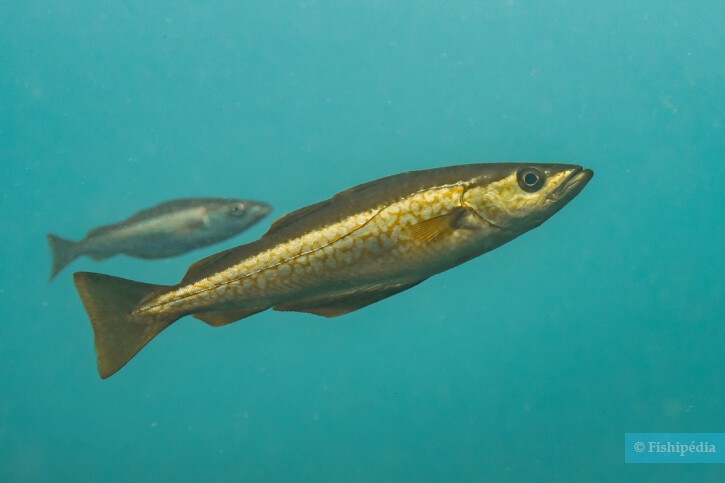The image features two fish swimming in a body of teal greenish-blue water. In the foreground, a sleek golden fish with a shimmery texture and a brown eye gracefully swims upwards towards the top right corner. This larger fish displays a striking golden animal print pattern. Just to the left and slightly above, a smaller fish appears more muted and less detailed, with a silvery greenish-blue hue that lightens in the middle of its body, blending subtly into the background. The serene aquatic scene is punctuated by a small blue banner in the lower right-hand corner that reads "© Fishipedia" in lighter blue letters.